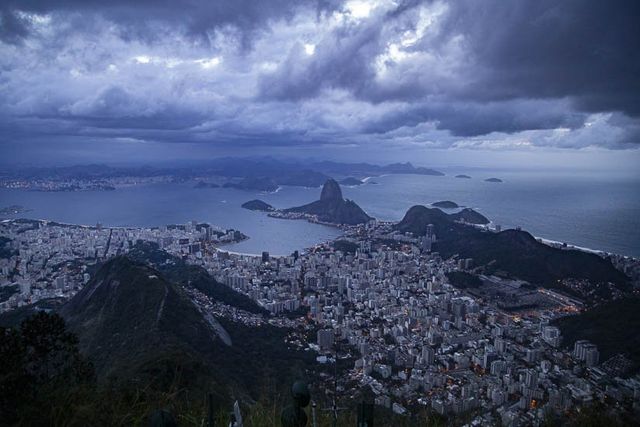This image presents a high-angle view, possibly from a mountain, capturing a cityscape under a stormy night sky. The predominant hue is a dark blue, likely due to a blue filter or color overlay. The foreground features rugged cliffs and rock outcroppings, suggesting a rocky coast with no visible beach. Below, there are numerous tall buildings, including skyscrapers likely serving as office and apartment structures, indicating a bustling coastal city. The ocean appears calm, with little wave activity. In the distance, several islands are visible; one large island on the left and three smaller ones on the right, the latter merely tiny blips against the horizon. Above, storm clouds dominate the sky, dark gray and lit sporadically by flashes that could be moonlight or lightning, hinting at impending heavy rain. The overall scene, with its dramatic clouds, tranquil ocean, and rugged landscape, evokes the atmospheric beauty often associated with places like Scotland or Ireland.